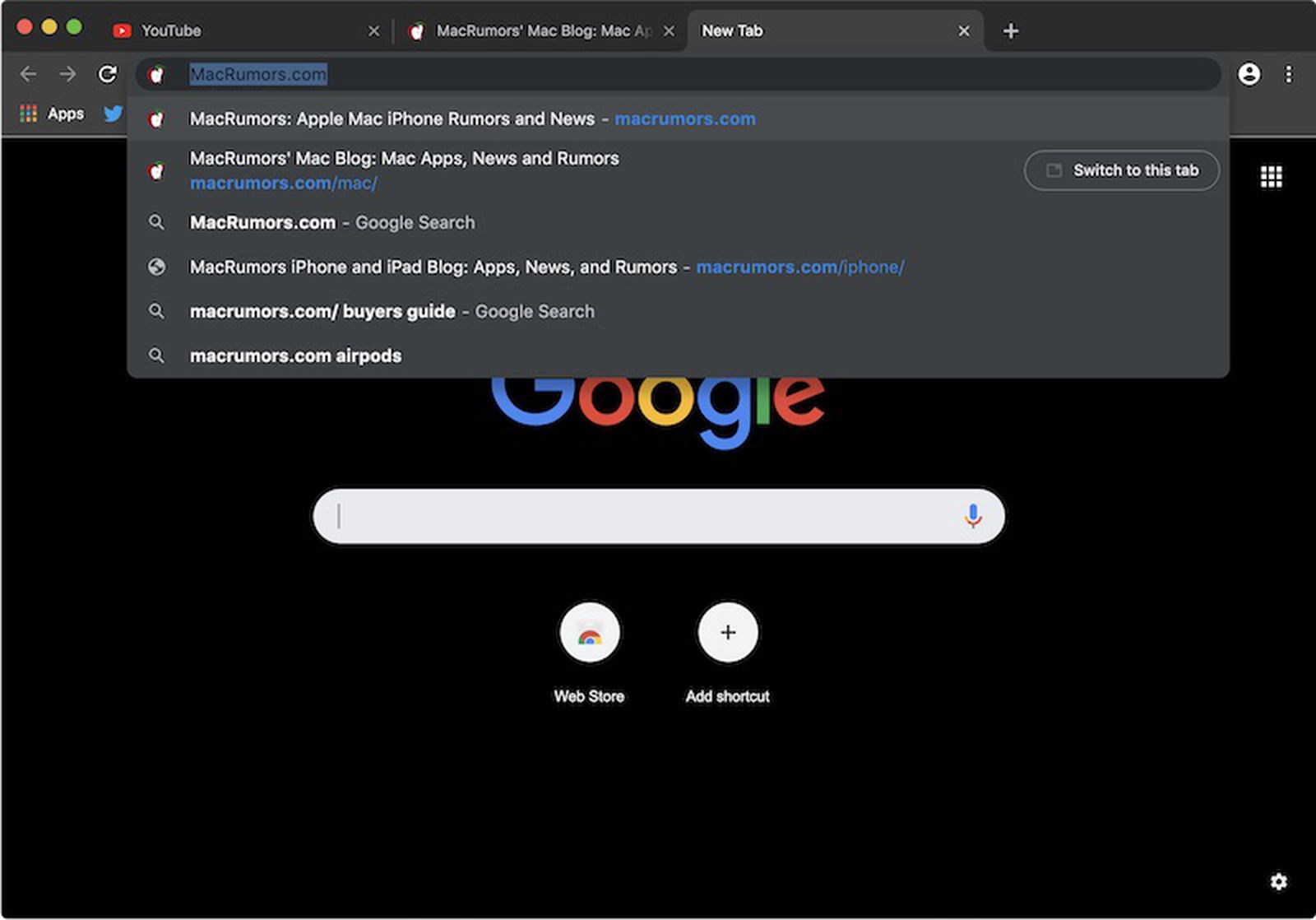The image depicts an Apple computer screen with the Safari browser open in dark mode, indicated by the gray background. Multiple tabs are visible, including YouTube, MacRumors, MacBlog, and an additional new tab. The user has searched for "MacRumors.com" in the address bar, yielding six different search results: "MacRumors.com," "MacRumors.com/mac," "MacRumors.com/google-search," "MacRumors iPhone and iPad Blog - Apps, News, and Rumors," "MacRumors.com/buyer's guide," and "MacRumors.com/AirPods." The current tab displays the Google start page, where nothing has been typed into the search bar. The page also features shortcuts like the Google Chrome Web Store and an "Add Shortcut" button.